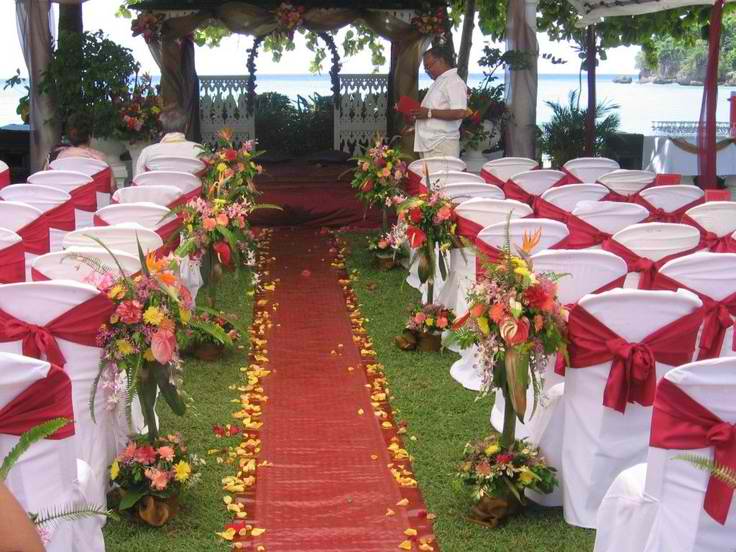This image captures a picturesque outdoor wedding venue. Central to the scene is a narrow red path, likely covered with a fabric runner, bordered by lush green grass sprinkled with a scattering of red and yellow flower petals. Alongside this path, every few feet, sit large vases overflowing with a variety of flowers. Flanked on either side of the path are rows of white folding chairs adorned with white covers and accented by elegant red ribbons tied at the back. To the left of the path, two rows of these chairs are visible, while to the right, there are three rows. 

At the end of the red aisle is a flat ceremony area, fronted by two sturdy wooden beams supporting a crosspiece adorned with floral arrangements. Beyond this structure, a small arch covered in greenery stands between two sections of white fencing, framing the backdrop. Gentle greenery blankets the arch, adding a touch of natural charm.

A man, dressed in a collared, button-down white shirt with a gold watch on his left wrist, stands to the right of the aisle. He appears engaged in reading from a red book, adding a solemn touch to the preparations. Behind him, a tall tree stretches into the background, and a large body of water glistens at the horizon, completing this serene and elegant setting.